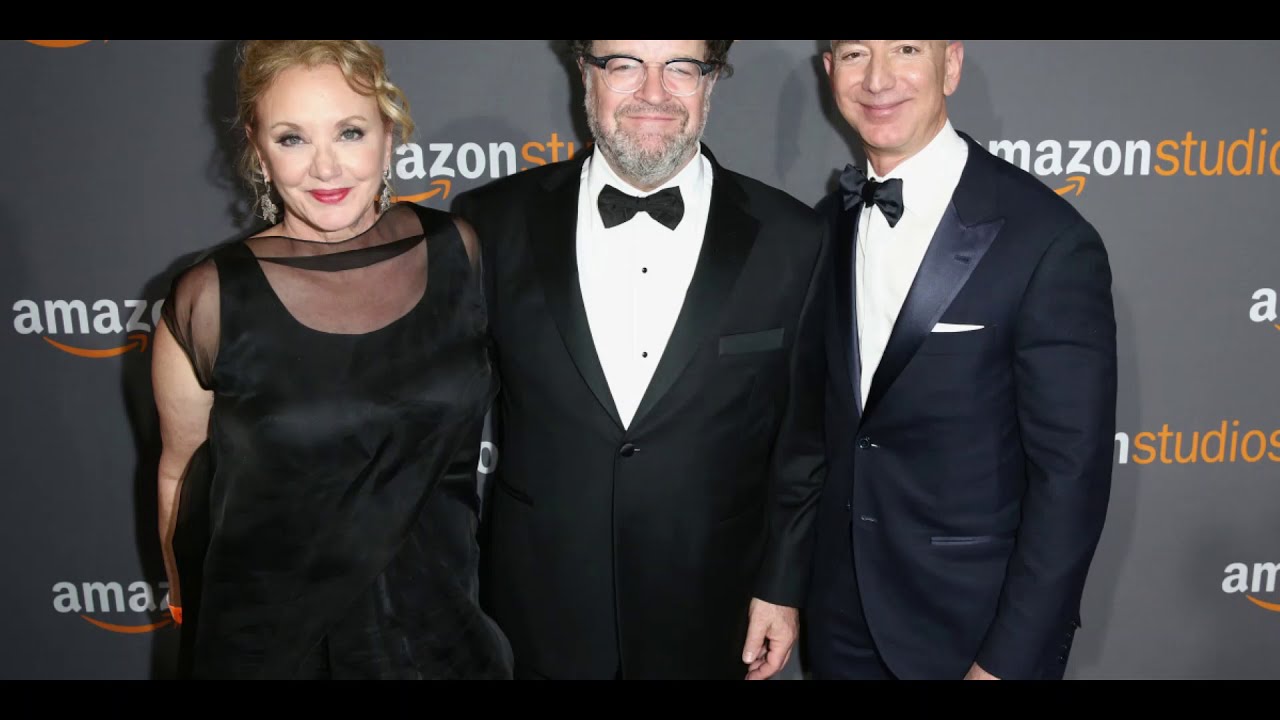In this photograph, three people are posing closely together in front of a gray backdrop emblazoned with the Amazon Studios logo in white and yellow text. On the right side stands Jeff Bezos, identifiable despite the photo's crop cutting off the top of his head. Bezos is dressed in a black tuxedo, paired with a white dress shirt and a black bow tie. In the middle, there's a heavier-set man with a gray beard and mustache, donning a black tuxedo and glasses. He appears to have his left arm around the woman on the left, whose long, wavy blonde hair, blue eyes, and red lipstick complement her smile and prominent cheekbones. She wears a black satin dress with short mesh sleeves and potentially translucent, lacey detail at the chest area. The elegant trio appears to be attending a premiere event, suggested by their formal attire and the polished backdrop.